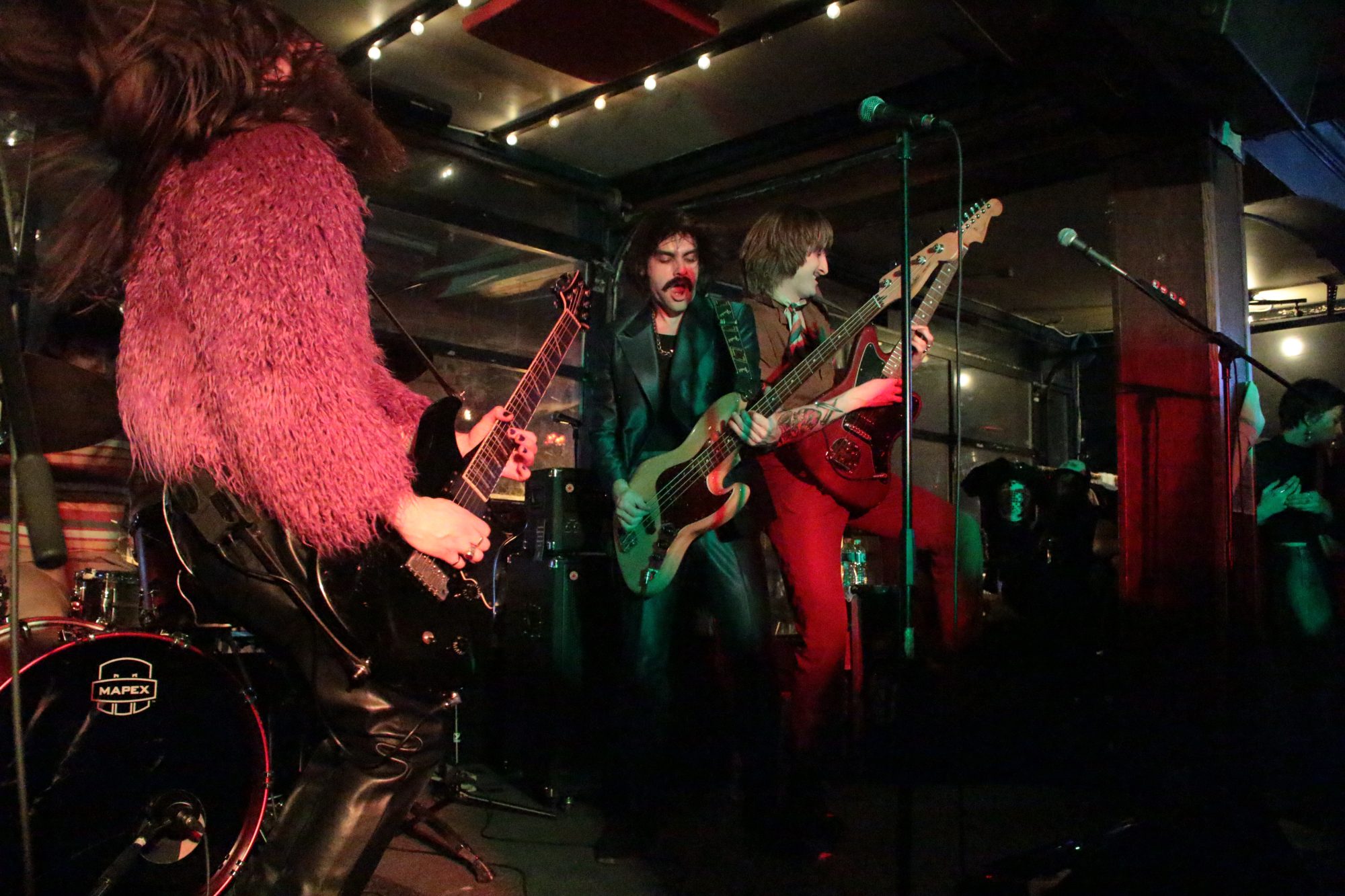The photo captures an intense performance by a three-member band on stage. At the center, two men stand shoulder to shoulder. The man on the left, with black hair and a black mustache, is energetically singing with his mouth open. He dons a black leather jacket and black leather pants while strumming a tan guitar. The man to his right stands out in tight red pants and a brown jacket or vest, holding a red guitar. He has long brown hair and wears a tie, his expression focused and intense.

To the left, closest to the camera, is a woman with her back partly turned. She wears black leather pants and a very furry pink long-sleeve shirt, her long brown hair cascading down as she plays a black guitar. Behind her, a drum set is visible. Surrounding the stage are various microphones, capturing the essence of their live concert. Off to the right, some people can be seen loitering, absorbed in the band's passionate performance. A forest green light bathes the scene, enhancing the vibrant atmosphere of the stage.